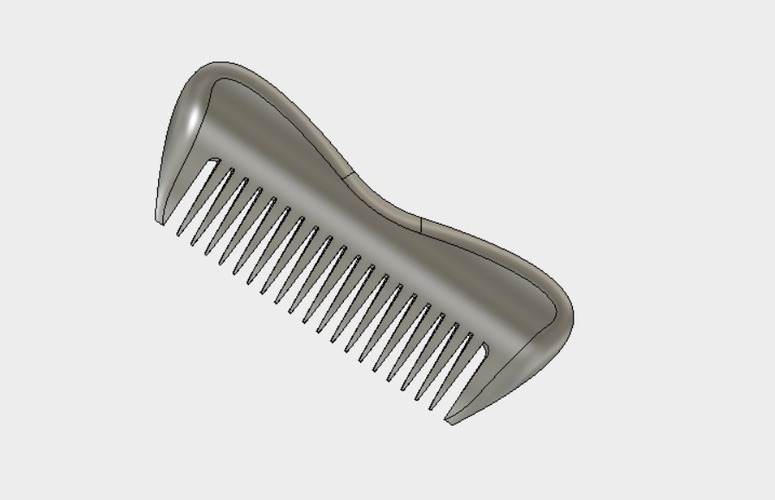This image features a computer-drawn, futuristic comb set against a light gray background. The comb, which serves as the central focus, is rendered in a variety of gray tones to add depth, dimension, and a touch of realism, including darker grays for shadow and a light sheen of white for highlights. Unlike traditional combs, this one is designed with a wavy, contoured handle that provides a comfortable grip to prevent it from slipping during use. The comb is oriented diagonally, enhancing its dynamic, three-dimensional appearance, as if it were modeled for 3D printing. It features twenty evenly spaced, sharp teeth, with the outermost teeth being wider to facilitate easier hair combing. The overall design appears quite unique and futuristic, diverging from the typical straight-edged designs one might expect.